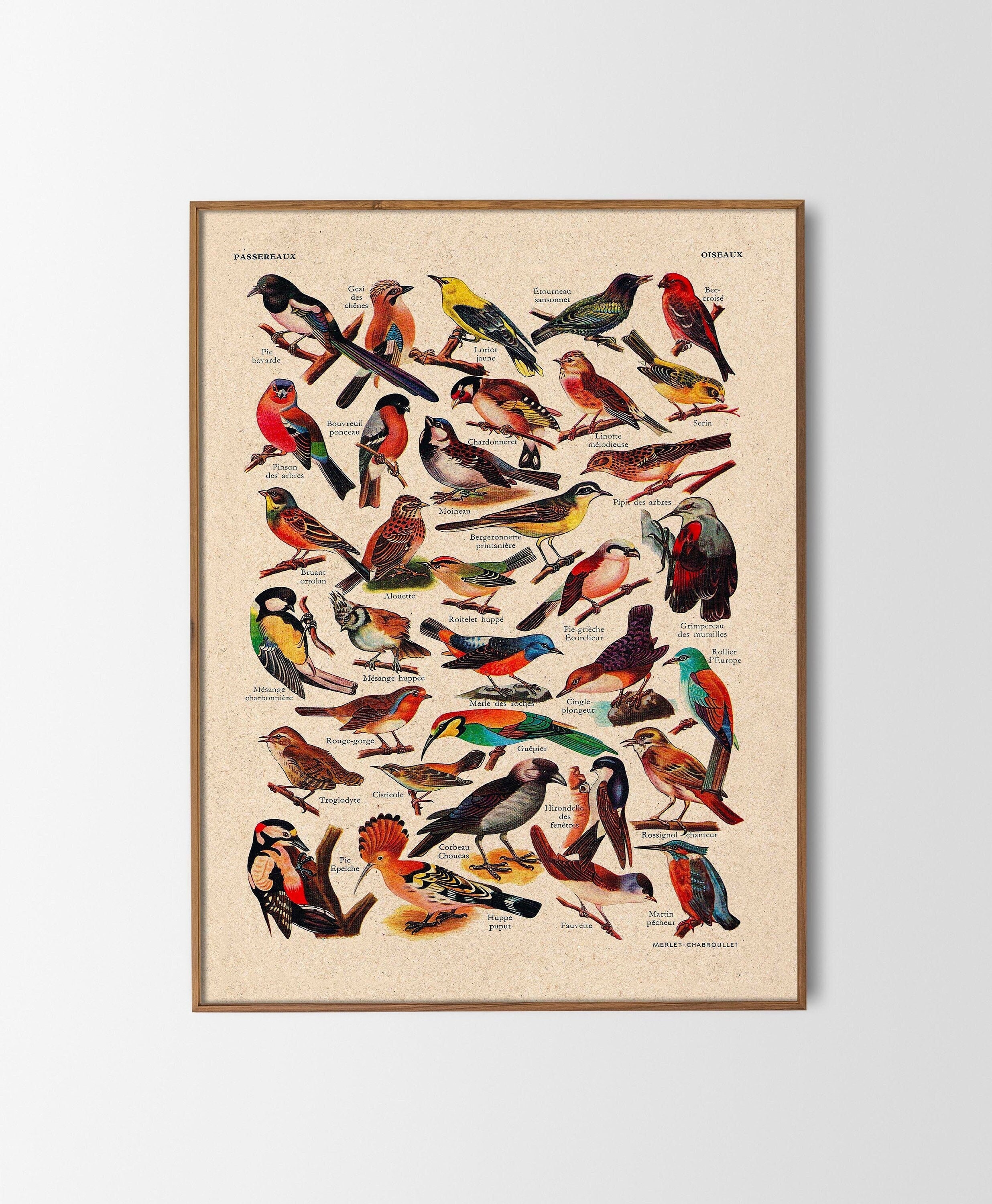The image depicts a framed art piece resembling botanical drawings, but featuring various bird species instead. The thin frame, which is either gold or medium brown, hangs on a stark white wall with no other elements visible. The artwork is meticulously detailed, showcasing approximately 25 birds of different shapes, sizes, and vibrant colors, including reds, blacks, yellows, blues, and greens. The birds are arranged almost in rows and columns against a beige, sandy-colored background, making their outlines and intricate features stand out. Each bird is accompanied by a small label that likely names the species, although the text is too small to read. The composition and detail reflect the beauty and diversity of the avian world.